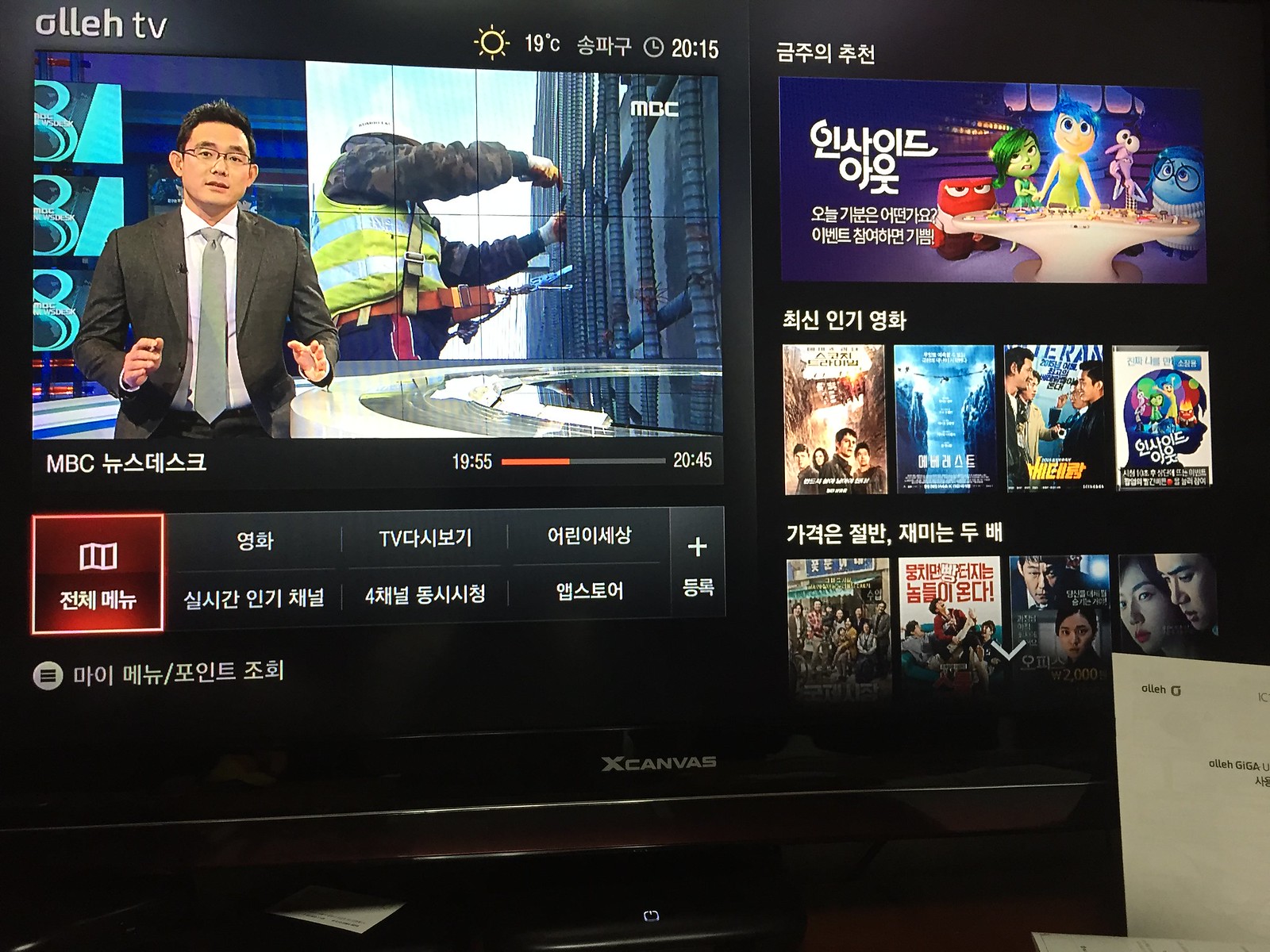This photograph captures a television or computer screen displaying content primarily in Korean. At the top of the screen, the brand "OLLEH TV" (spelled O-L-L-E-H) is visible. In the upper left corner, the interface includes a small depiction of a sun icon accompanied by the temperature and time. Central to the image is a male newscaster, potentially wearing glasses, making hand gestures. Behind him, a background video shows a construction worker handling steel. The lower part of the screen is divided into several boxes featuring text in an Asian script, likely Korean, which are not legible to an English reader. These include various shades, with one notable red box outlined in red. On the right side, there appears to be a selection of video options for movies or TV shows, including what looks like a cartoon. A piece of paper is partially visible at the lower right corner of the photograph, adding to the detailed yet complex visual arrangement.